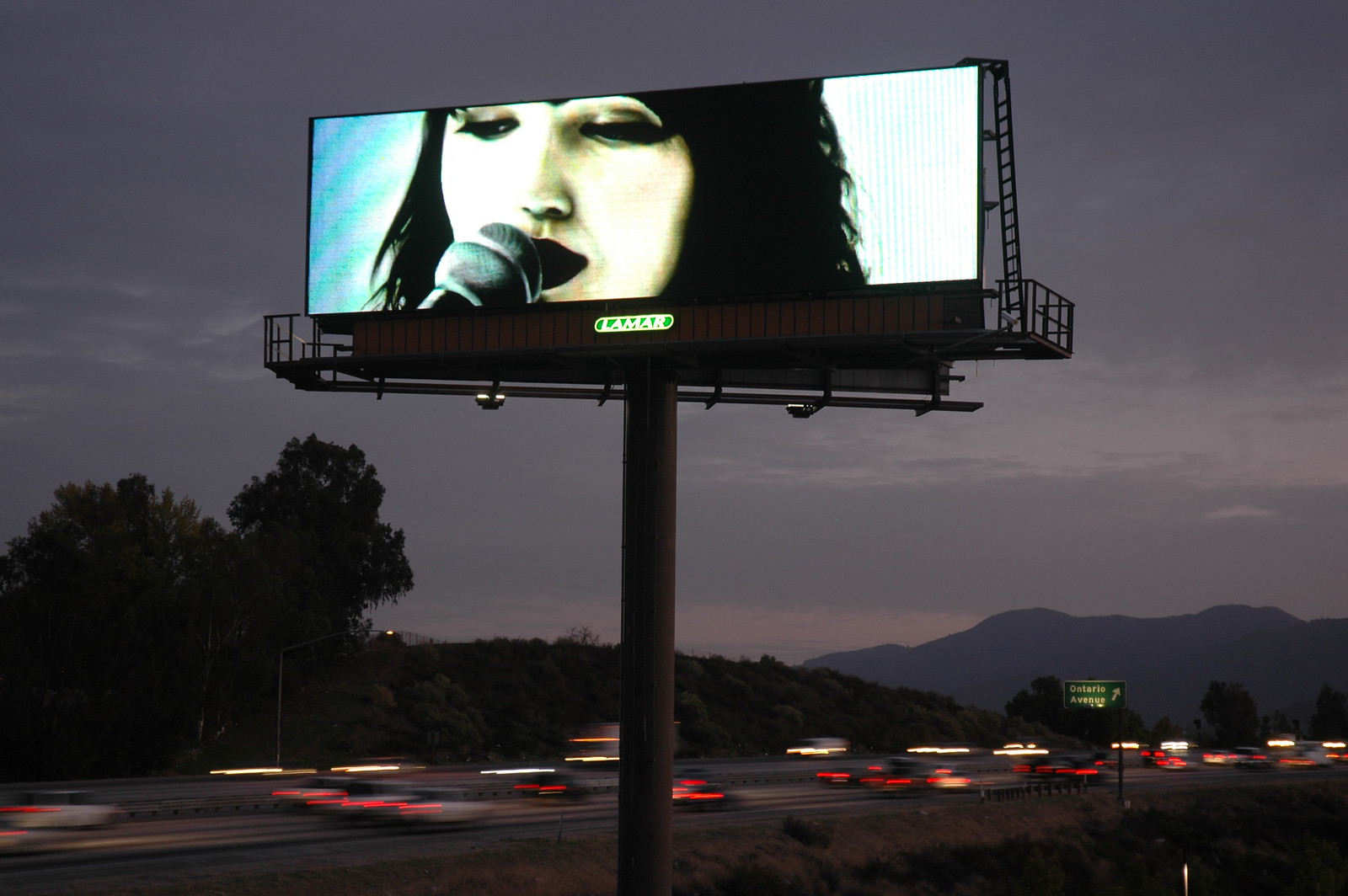In this color photograph, taken at twilight or possibly very early morning, a large, illuminated billboard dominates the center of the image. The billboard features a high-contrast black and white image of an attractive woman with dark, possibly goth-inspired makeup, characterized by dark hair, semi-closed eyes with heavy mascara and eyeliner, and very dark red lipstick. She holds a microphone close to her lips, suggesting she's a singer or performer.

The backdrop reveals a dusky sky transitioning from dark blue to violet, hinting at either impending nightfall or the last moments of sunset, with faint pink hues lingering over distant mountains. Below the billboard, the photo captures a busy freeway with the red blur of taillights on one side and the blur of headlights on the opposite, indicating the motion of numerous cars. Amid the traffic, a sign reading "Ontario Avenues" can be seen, with white writing on a green background, pointing right.

To the left side of the image, the outlines of leafy trees are discernible, accentuating the natural elements amidst the urban environment. To the right, dark blue hills frame the scene, enhancing the overall composition of the landscape. An embankment full of grass slopes down from the road, tying the thematic elements of nature and city life together in this evocative, slightly out-of-focus snapshot.